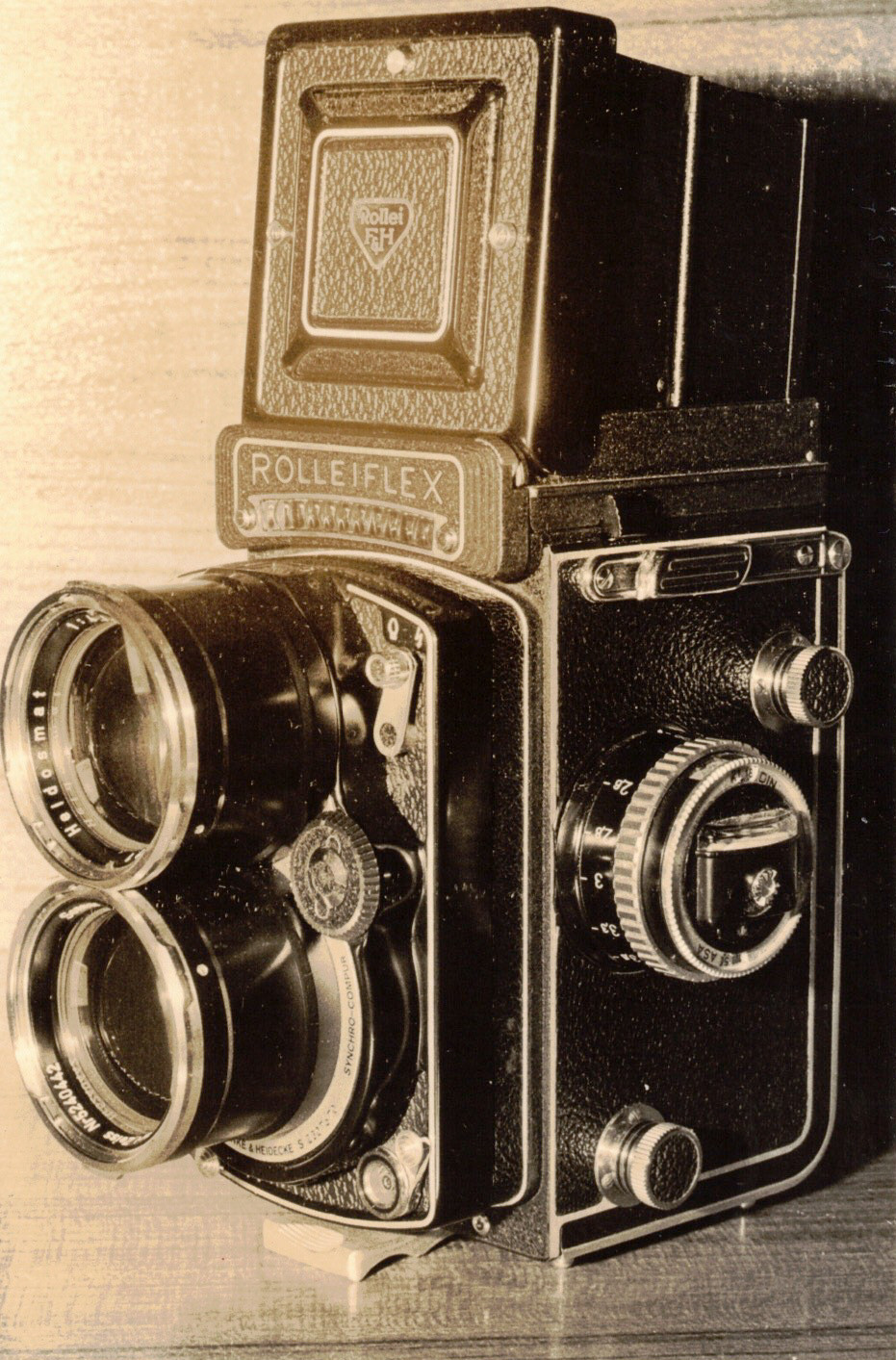The image features an antique Rolleiflex camera with a design characteristic of the 1920s. This dual-lens camera, arranged with one lens on top of the other, is oriented to the left, with the left side brightly lit and the right side in shadow, indicating a light source from the left. The camera, primarily black with a hazy brown tone overlay in the photograph, sits on a shiny, possibly ceramic, tabletop or a wooden shelf. Just above the lenses, the brand "ROLLEIFLEX" is prominently displayed on a small rectangular label, accompanied by an additional serial number. The camera's top section is a square box-like structure that you'd look down into while the bottom section retains a sturdy box form. Distinct knobs and dials, including a round calibrated dial with visible numerals, are situated on its side for adjusting settings. Despite some of the labels being difficult to decipher in the current lighting, the overall intricate design captures the essence of a classic photographic tool.